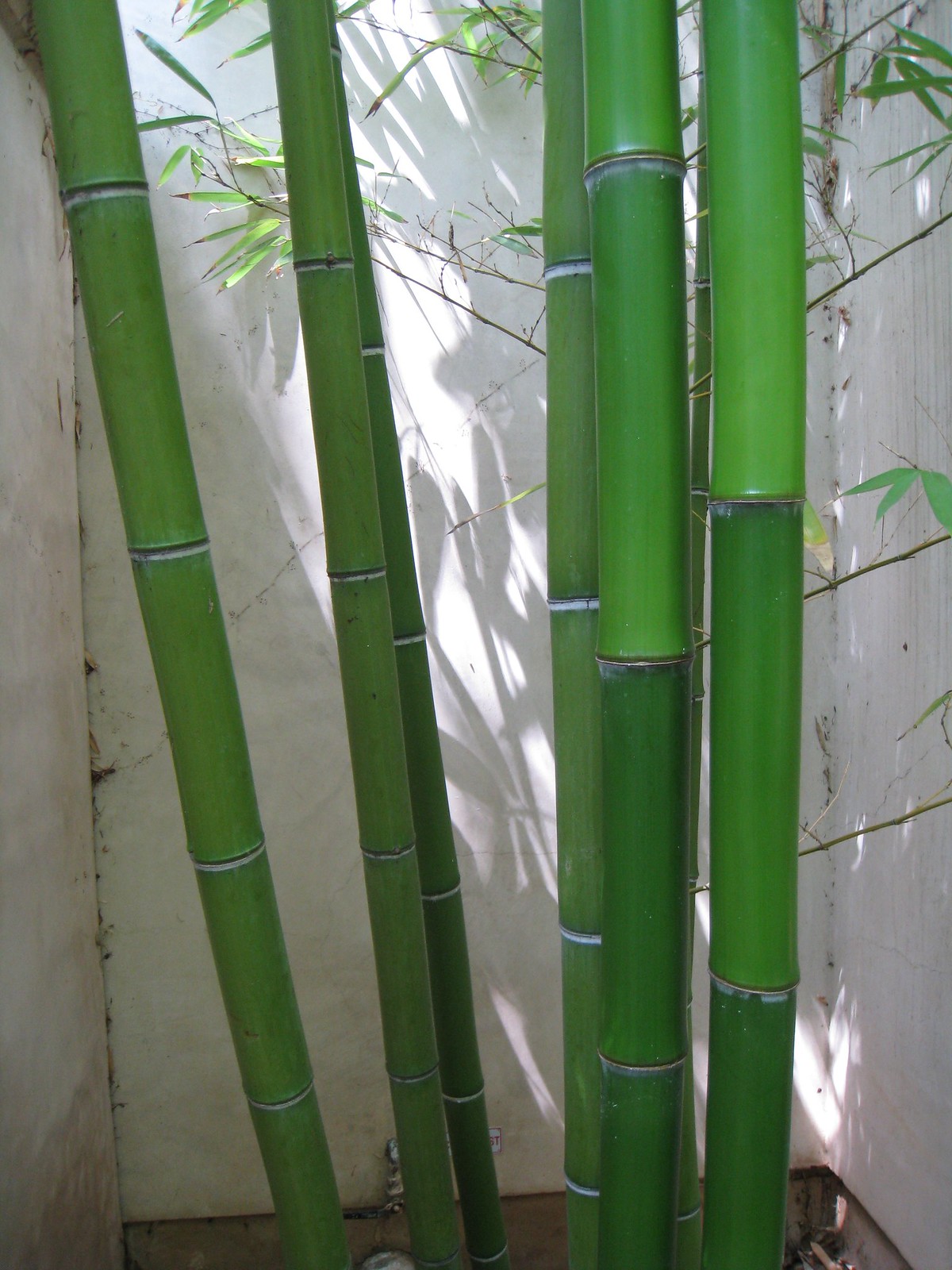In this image, we observe a small, enclosed space characterized by three white walls forming a tight square area. The floor appears to be composed of a rough concrete texture, with earnest hints of nature as a tiny plant peeks through the cracks. The focal point, however, is a striking presentation of tall, vibrant green bamboo shoots, numbering between six and seven. These shoots are interspersed with thin branches and delicate green leaves. The bamboo sections feature subtle variations in color, with some parts being slightly darker and displaying horizontal stripes with patches of white. The setting hints at being an outside enclave, accentuated by shadows cast by the bamboo under sunlight, adding depth and dimension to the stark white surroundings.